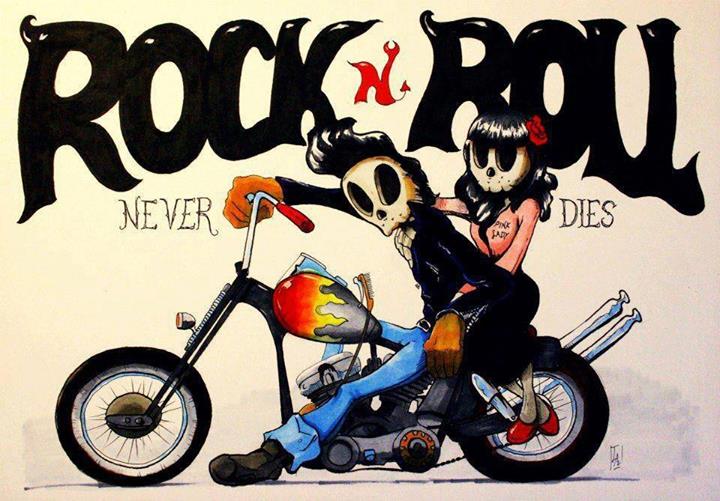The rectangular poster features a vivid cartoon drawing of two skull-faced characters on a stylized motorcycle, projecting a distinct punk attitude. Positioned centrally, the motorcycle, adorned with red and yellow flames on its black gas tank, has silver exhaust pipes and metal silver-spoked wheels. The male rider, with a pompadour hairstyle, sports a leather jacket, cuffed blue jeans, and black boots. His female companion, with long black hair in a Betty Page style and a red rose, wears a pink button-up jacket labeled "Pink Ladies" and red heels. Both characters with skeletal faces exude a greaser vibe. 

At the top of the poster, large bubble text reads "Rock In Roll," with "Rock" and "Roll" in black and "In" in red, complete with devil horns and a tail. Below, in elegant script, the words "Never Dies" are split, positioned beneath "Rock" and "Roll" respectively. The background starts as light yellow on the left, fading to a grayish hue on the right, emphasizing the bold, edgy aesthetic of the image.